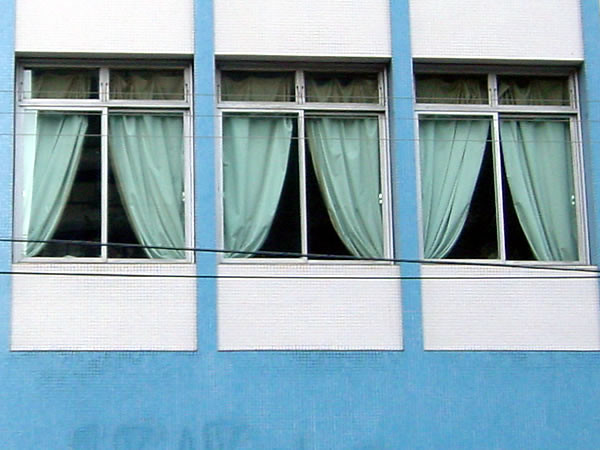This color photo captures a close-up of the front of a building featuring three aluminum-framed windows, highlighted by a combination of baby blue and white paint. The walls of the building are primarily painted baby blue, with white trim framing the windows at the top and bottom. Each of the windows is divided into four panes: two small transoms at the top and two larger panes below, likely functioning as sliding windows. The windows are closely set, separated by narrow baby blue columns, while the top and bottom portions of the wall surrounding the windows are painted white. Visible from the slight upward perspective of the photo are the backs of shimmery, white, blackout or opaque drapes, creating swag shapes where they have been drawn together. Additionally, an electrical or phone wire crosses the scene, contributing to the dated aesthetic of the building. Despite the bright colors, the structure's style hints at an older construction, giving it a somewhat run-down yet charming look.